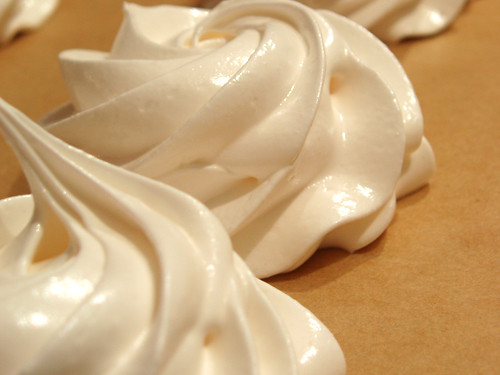The image features an extreme close-up of several perfectly formed, creamy white mounds of soft ice cream positioned in a neat row on a shiny, sand-colored surface resembling parchment paper. The ice cream, likely vanilla, exhibits a silky texture and is freshly dispensed from a machine, with each mound crowned by a small, elegant swirl. While the photograph highlights primarily one and a half mounds clearly, additional mounds are partially visible in the background, with some just slightly cut off, maintaining their shape and showing no signs of melting. The intricate lines from the dispensing machine are evident on the mounds, emphasizing the pristine and glossy finish of the ice cream, making it appear even more appetizing.